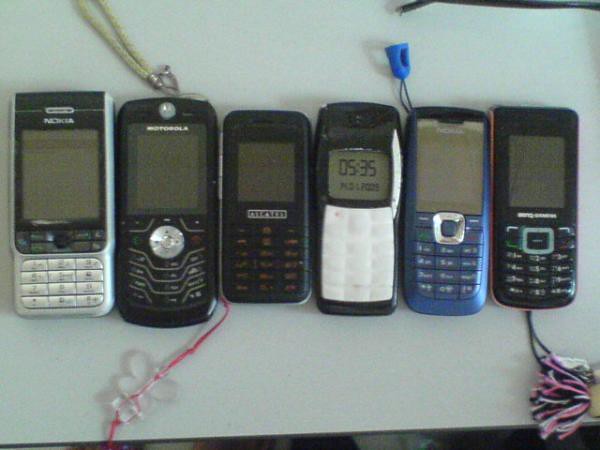The image is a color photograph featuring six old cell phones arranged horizontally in a row against a light gray or white tabletop background. Starting from the left, the first cell phone is a Nokia with a black top and silver bottom. Next is a black Motorola phone with a white lanyard attached to it. Following that is a small black cell phone, brand unclear. The fourth phone is black with a white keypad, displaying the number 535 on its screen. The fifth phone in the sequence is blue and turned off, resembling a track phone, while the last phone is black and also turned off. Some of the phones feature decorative attachments like keychains or ribbons, with one having a pink ribbon adorned with a translucent butterfly bead and another with a pom-pom made of pink, white, and black yarn.